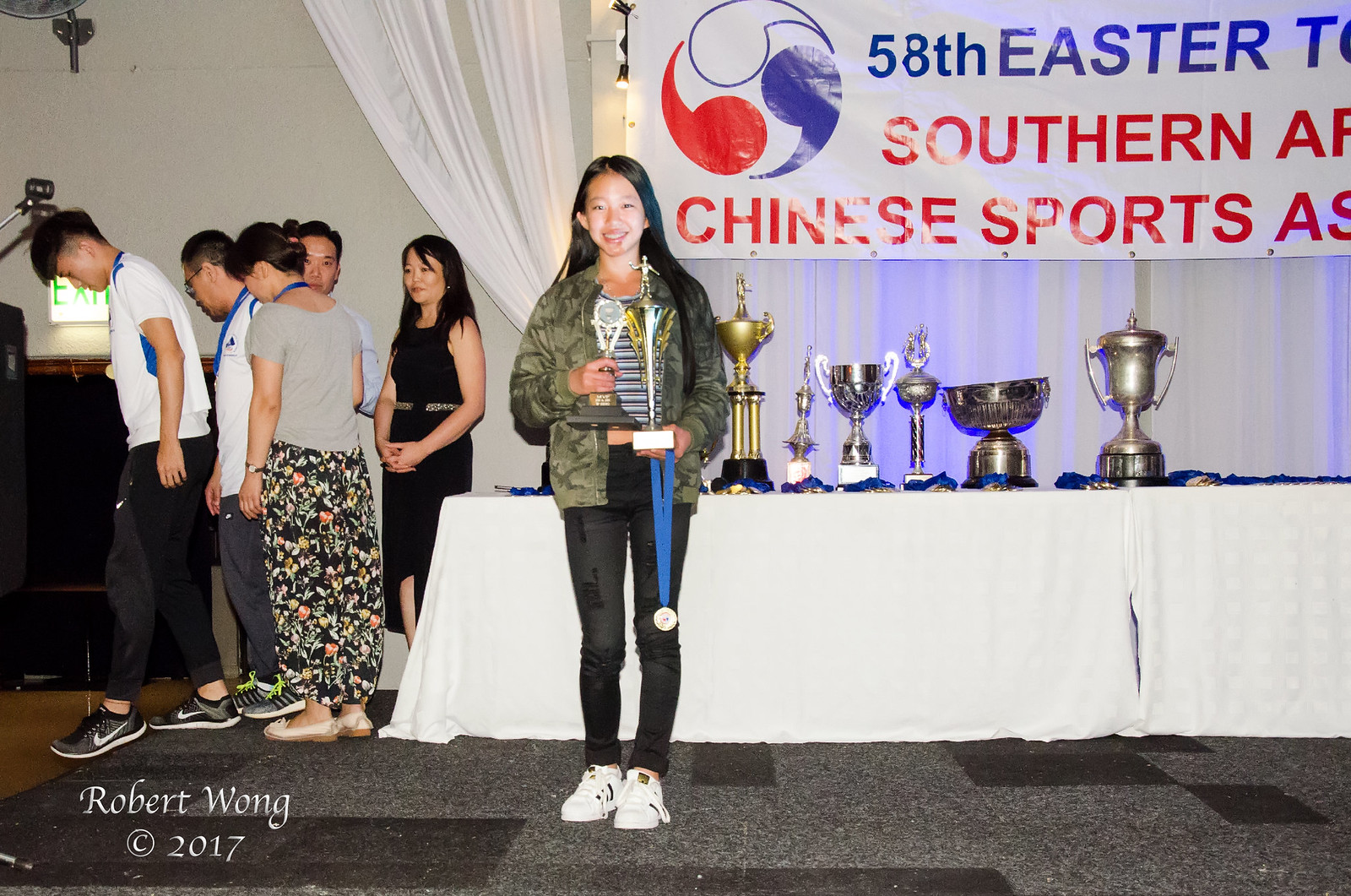In the image, a smiling teenage girl with long black hair, dressed in a camo jacket, black and white striped shirt, black pants, and white tennis shoes, stands proudly holding a small silver trophy, a larger gold cup-style trophy, and a medal. She is at the forefront of what appears to be an award ceremony for the 58th Easter Southern Chinese Sports event, as indicated by the partially visible poster and logo in the background, which features red, white, and blue colors and a ball. Behind her, a table draped with a white cloth showcases at least six additional trophies and numerous medals, suggesting significant recognition of achievements. To her left stands a Chinese woman in a sleeveless dress, and behind them, under a curtain, are five individuals, likely a mix of adults and children, all adorned with medals. The image is credited to Robert Wong, © 2017.